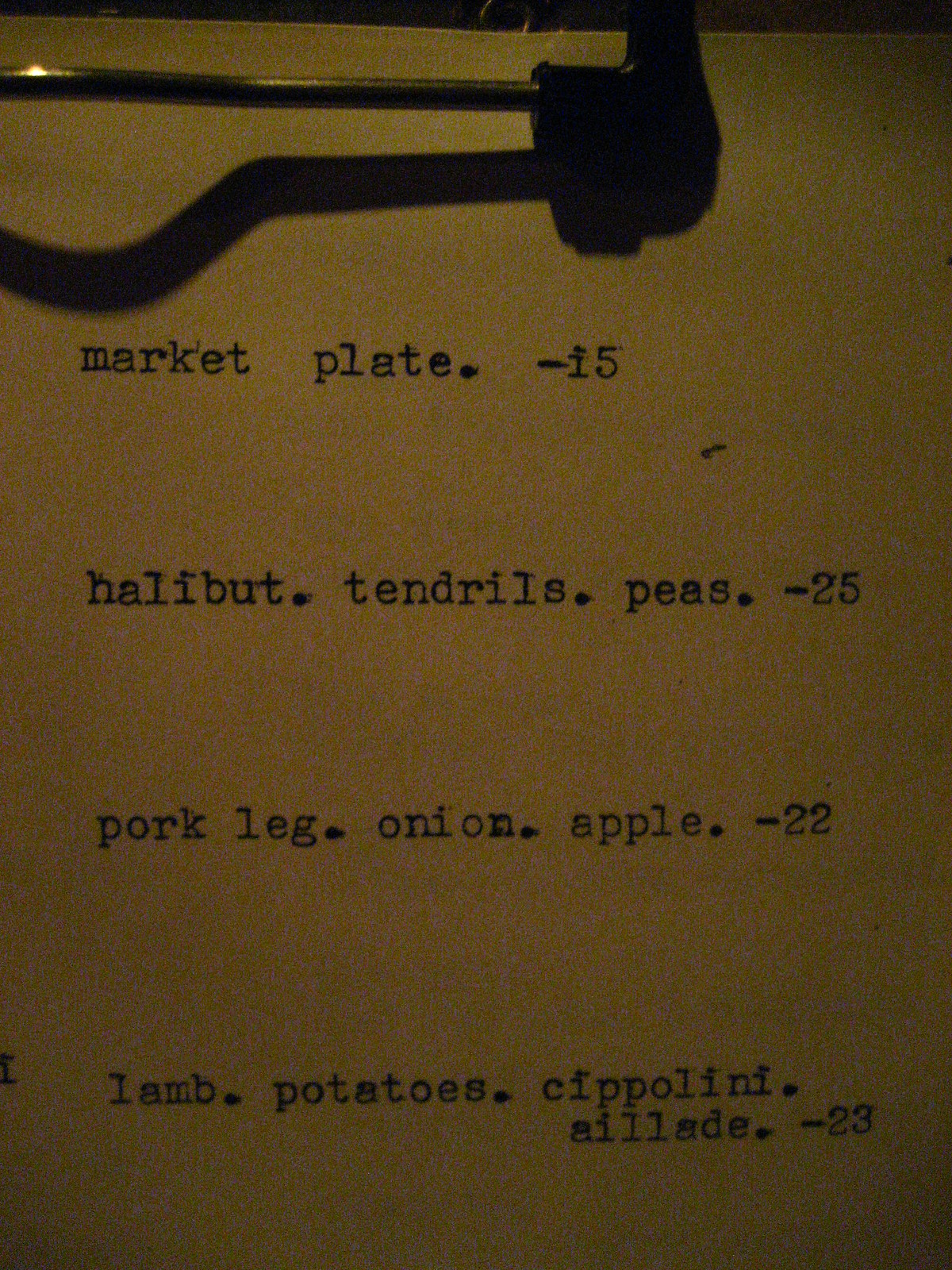The image captures a nostalgic moment featuring a close-up of a manual typewriter at work. The scene is dimly lit, evoking a sense of antiquity and focus. At the top of the image, we observe a metal clip – part of the typewriter's mechanism – firmly securing a sheet of paper. The clip casts a subtle shadow on the paper, enhancing the vintage ambiance.

The typed text on the paper stands out clearly amid the subdued tones. The words are arranged in a list format, beginning from the upper left corner and continuing downward in neat alignment. The text is as follows:

1. MARKET
2. PLATE
3. I5
4. HALIBUT
5. TENDRILS
6. PEAS
7. 25
8. PORK LEG
9. ONION
10. APPLE
11. 22
12. LAMB
13. POTATOES
14. CIPOLLINI
15. I LATE
16. 23

This image transports the viewer back to a time when typewriters were the epitome of modern technology, capturing the essence of a bygone era defined by the tactile click-clack of metal keys and the crisp imprint of inked typeface.